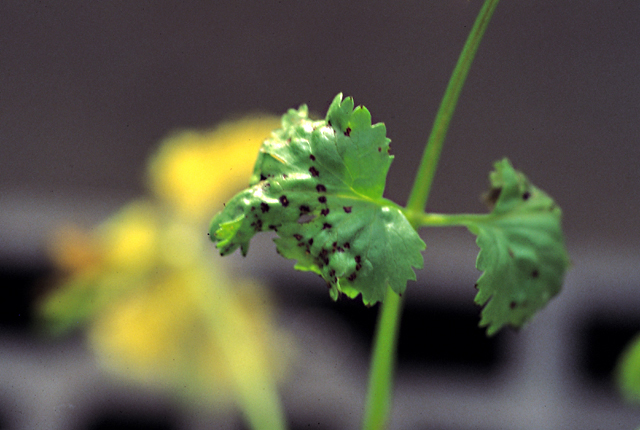The image is an extreme close-up of a bright, lime green plant stem with two symmetrical and slightly curved leaves branching out from either side at the center. The leaves, possibly from a cilantro or parsley plant, exhibit an irregular, serrated edge and are dotted with black specks, suggesting disease or infestation. The background is heavily blurred, featuring indistinct patches of yellow, possibly from another plant or flowers, as well as some gray and dark brown tones. The main focus is sharply on the vivid green leaves and stem, creating a striking contrast with the out-of-focus and colorful backdrop.